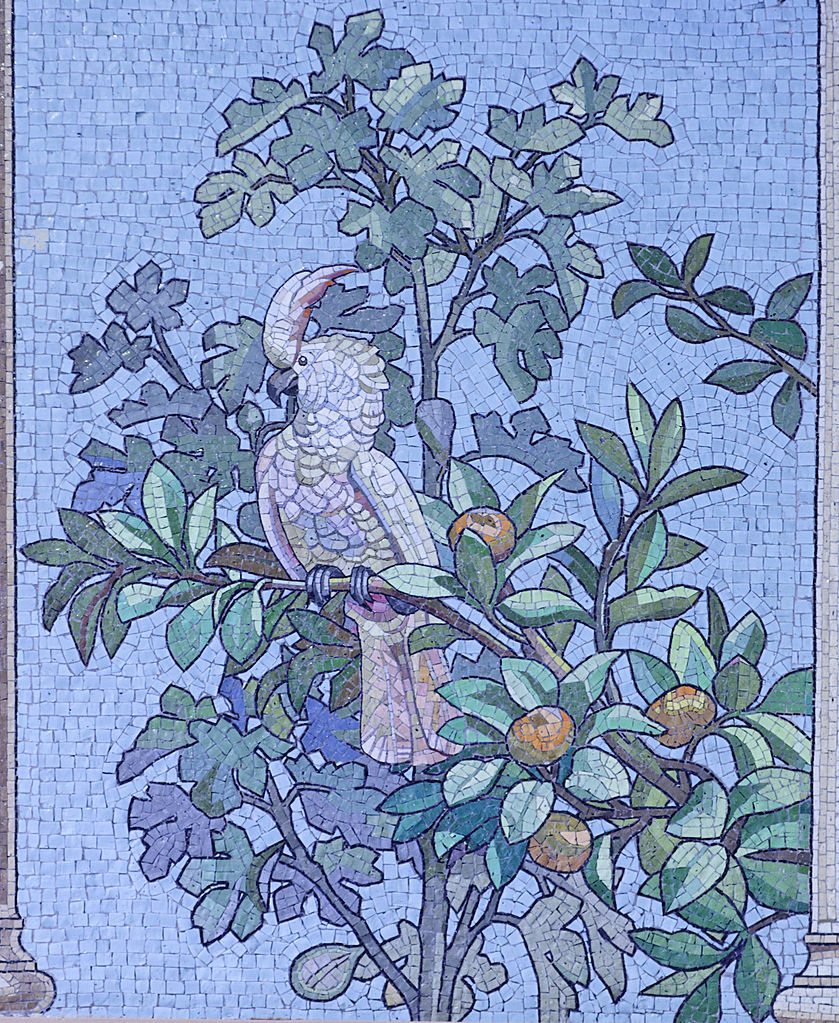This intricate mosaic painting depicts a serene scene centered around a white parrot perched on a fruit-laden tree. Comprised of numerous small, square and rectangular tiles, the artwork offers a meticulous rendering of vibrant details. The background is a rich, blue expanse made up of blue-colored tiles, suggesting a clear sky. Framing the composition, two light gray pillars are faintly visible on either side, indicating a classical architectural setting.

In the middle of this tile masterpiece, the parrot, with subtle pink and blue hues accenting its primarily white feathers and a dark gray beak, gazes thoughtfully to the left. The parrot is perched on a branch surrounded by green and bluish-green leaves, the hues becoming grayer beneath its perch. The tree also bears round, orange fruits, potentially oranges, persimmons, or mandarins, adding a pop of color and a touch of nature’s bounty. The overall scene is beautifully captured, blending organic elements with the structured geometry of the tile medium.